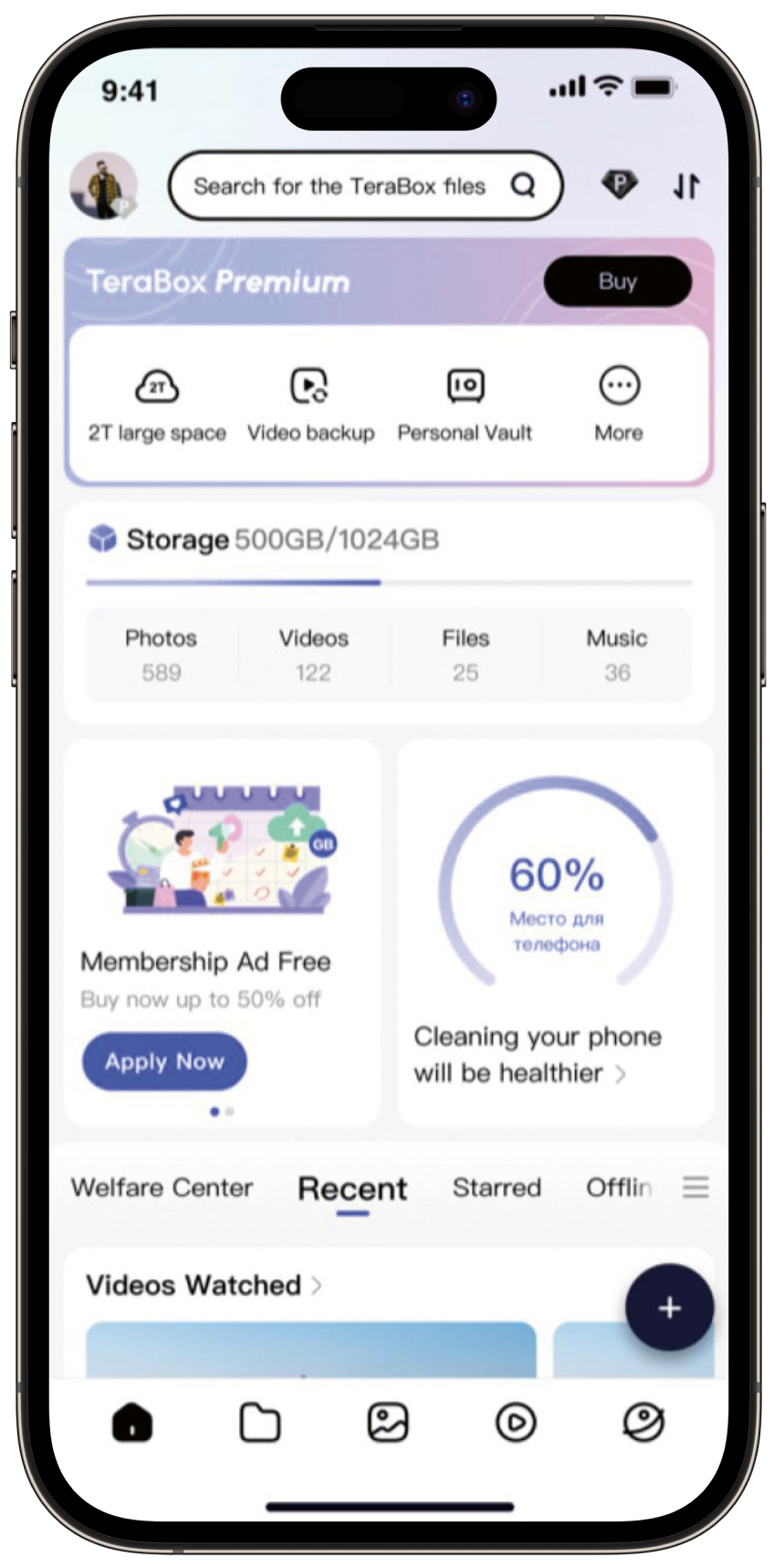At 9:41 AM, the phone display shows full signal, full Wi-Fi, and full battery. The user is wearing a jacket and is searching for TeraBox files using a magnifying glass icon labeled 'CP'. The screen displays options for TeraBox Premium, with a cloud icon indicating 2TB of storage space. Features listed include large space, video backup, personal vault, and more. A banner indicates 'Storage: 500GB / 1,024GB' with a blue progress line.

The categories are broken down as follows: Photos (589), Videos (122), Files (25), Music (36). An advertisement promotes an ad-free membership with up to 50% off, highlighted in a blue oval, and there is also a 60% off deal at McDonald's. A cleaning phone reminder is mentioned, implying a healthier device.

The screen features a black background with a centralized welfare center icon underlined. Additional icons include a star, an offline hamburger menu, and categories for watched videos. Several thumbnail images depict a blue sky. Icons present include a house, folder, picture icon, play button, and a planet icon with a dot. The biome graphic suggests a thematic gaming or environmental app, concluding the highly detailed description of the interface displayed on the screen.